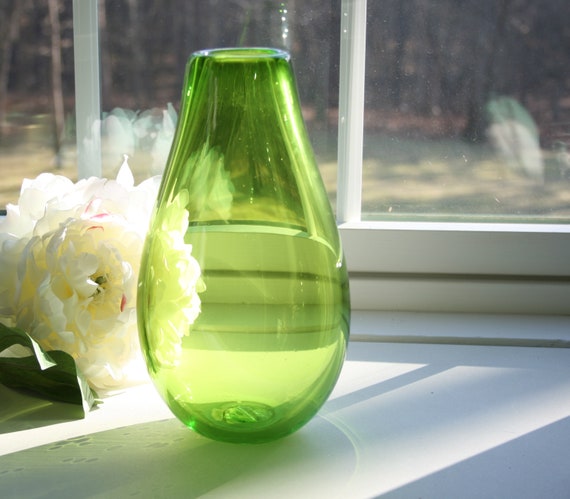A light green, oval-shaped glass vase sits empty on a white windowsill, bathed in sunlight. To the vase's right lies a large white flower, possibly a rose or peony, its numerous petals distinctively visible, along with a sliver of its green leaves. Through the window, blurred images of trees and a grass lawn merge into the edge of a forest, creating a serene backdrop. The sunlight reflects off the vase, illuminating the clean, white window frames and casting gentle shadows across the scene.